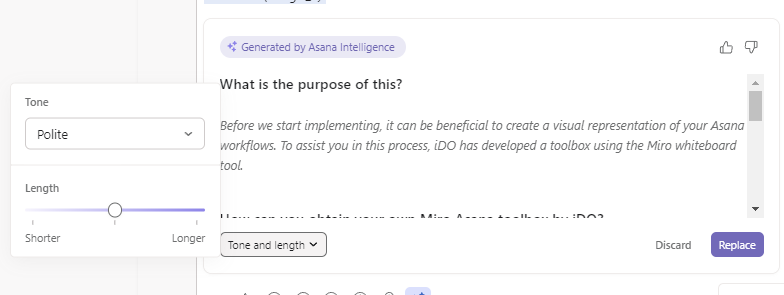The image displays the user interface for Asana Intelligence settings. On the left side, there is a pop-up menu labeled "Tone," which allows users to select the tone and length for text generation. The main section showcases a generated text block that begins with an explanation of the purpose and benefits of creating a visual representation of Asana workflows using the Miro whiteboard tool.

Below the generated text block are options to replace, discard, or modify the text based on the user’s tone and length preferences. The "replace" option is highlighted in a purple or blue color. Users can also upvote or downvote the response from Asana Intelligence to improve its accuracy and relevance. This interface highlights advanced features such as customizable tone and length settings, reflecting the continuous improvement of AI, which is both exciting and impressive.